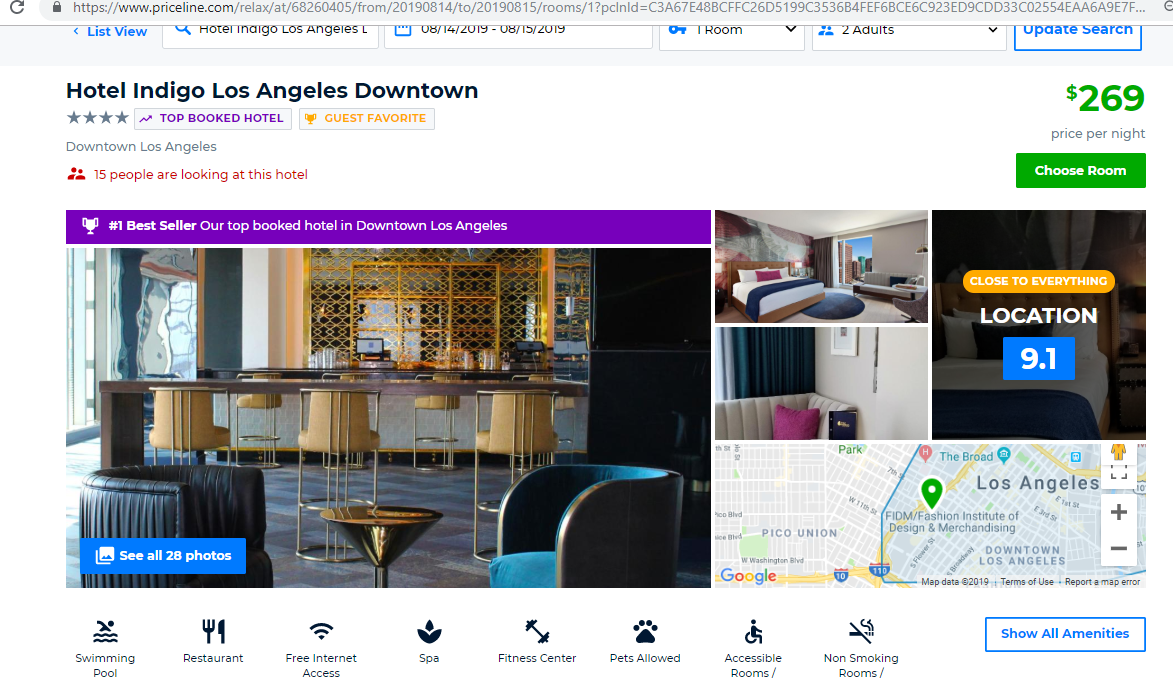**Detailed Caption:**

The image showcases the Priceline.com website open in a browser, focusing on the Hotel Indigo Los Angeles Downtown. At the top of the page, there are various tabs detailing the stay: "08-14-29 to 08-15-2019, 1 room, 2 adults." The "Update Search" button is prominently displayed in blue.

Below the tabs, the hotel's name appears twice: "Hotel Indigo Los Angeles," in a standard font at the top right, and as "Hotel Indigo Los Angeles Downtown," labeled as a 4-star hotel on the left. The hotel is distinguished as a "Top Booked Hotel" in purple and a "Guest Favorite" in yellow. The interface also indicates that "15 people are looking at this hotel," written in red text.

The nightly rate for the hotel is $269, displayed in green alongside a green "Choose Room" button. A picture of the hotel is presented on the left side, featuring an environment with brown, black, and blue chairs. Above the image, a purple banner announces, "Number One Best Seller: Our Top Booked Hotel in Downtown Los Angeles."

For more visual detail, there's a blue text link at the bottom left saying "See all 28 photos." Additional smaller images of the hotel are shown on the right side of the main photo, with one of them carrying the label "Close to Everything" on an orange background. A blue tag marks the location score as "9.1," and there's also a map at the bottom right corner.

Additional features and amenities listed at the page's bottom include icons for swimming pool, restaurant, free internet access, spa, fitness center, pets allowed, accessible rooms, and non-smoking rooms. There's also a blue link labeled "Show all amenities" for more information.